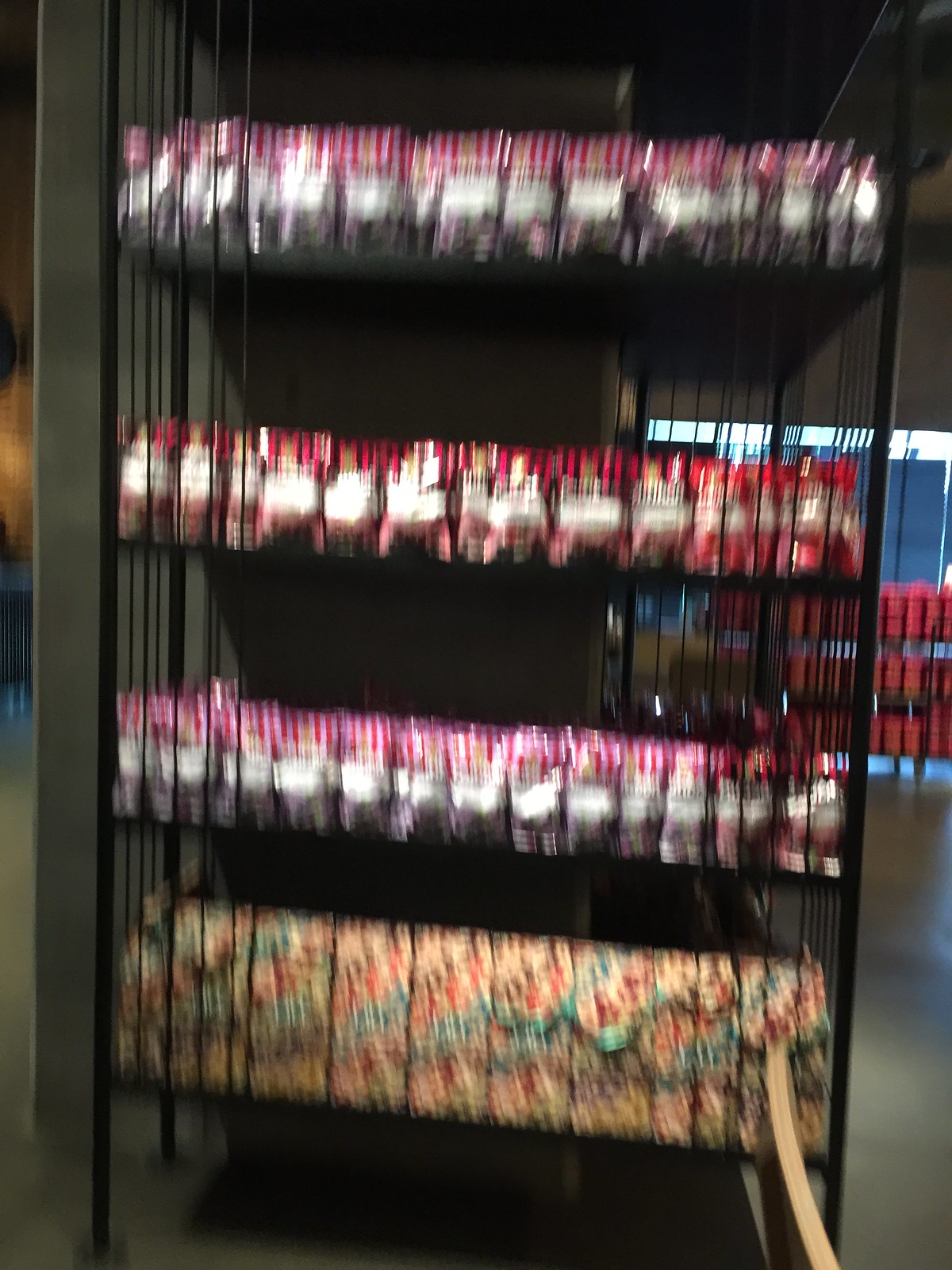The image features a vertically oriented, rectangular photograph with noticeable blurriness throughout. The focal point is a black metal rack that spans from the top to the bottom of the frame. This rack comprises four shelves, each stacked with food items. At the left side of the image, a dark green pole extends upward, parallel to the rack. The upper right portion of the background displays a green wall.

On the bottom shelf of the rack, there appear to be boxes of popcorn. The other three shelves above it contain similarly packaged items, potentially various flavors of candies. The second shelf from the bottom has items with a pink label at the top of their packaging, which matches the labeling on the topmost shelf. The third shelf from the bottom features goods with a red and black striped label at the top of each package. The floor beneath the rack is made of dark concrete. Toward the back left of the image, another rack can be seen, this one holding several red devices.